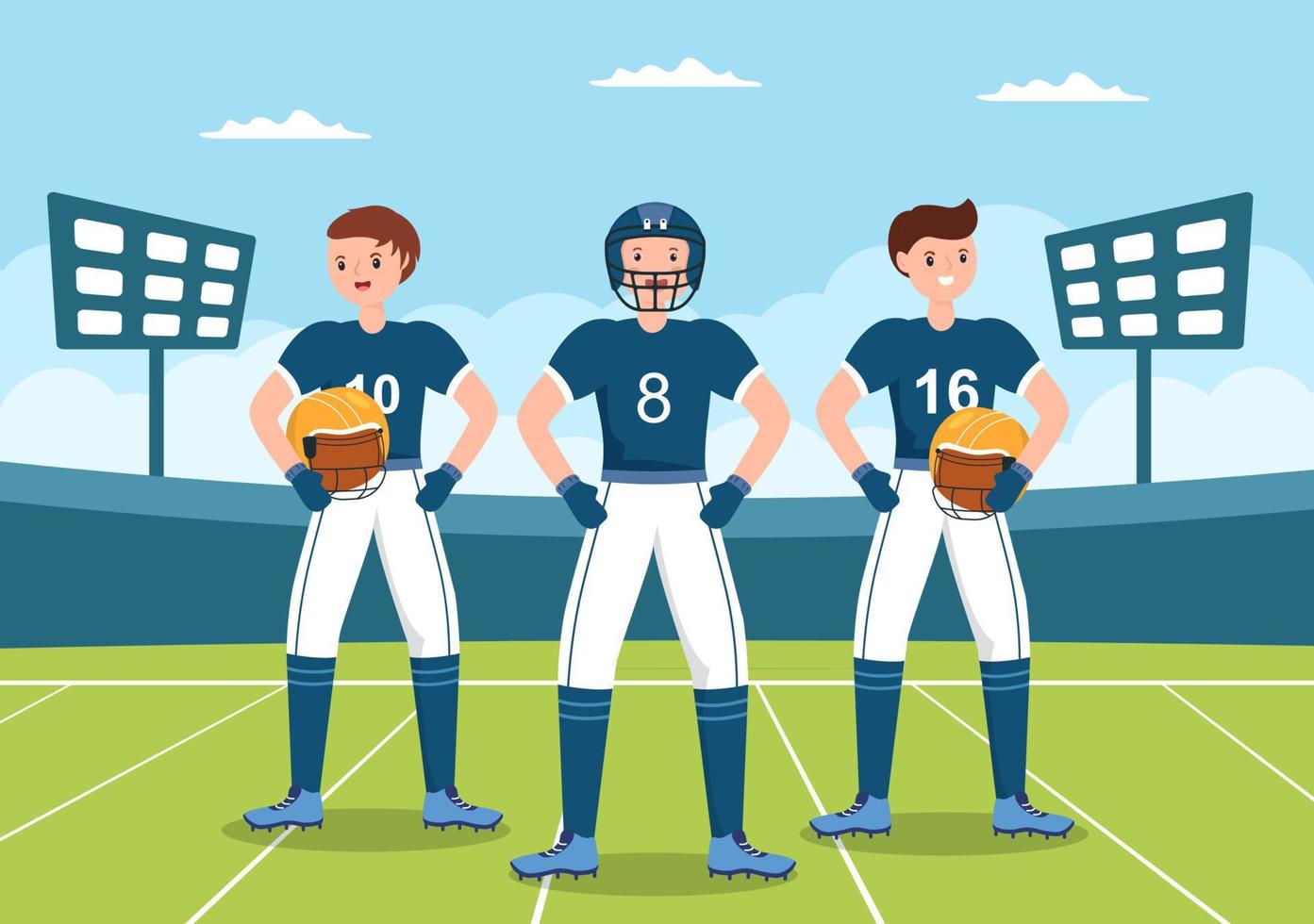The image is a detailed, computer-generated artwork featuring three animated football players standing on a green playing field marked with white lines. The background showcases a deep blue sky adorned with three distinct, white clouds and additional billowy clouds below in lighter shades of blue. The stadium is depicted in a matching dark blue color, and on either side of the field are blue and white scoreboards with blue poles, likely representing field or stadium lights.

The three football players are wearing dark blue jerseys with white numbers: one has the number 10, another number 8, and the one on the right has number 16. The players in the middle and left are holding yellow helmets with black face masks, while the player in the middle wears a dark blue helmet with a face mask. All the players have bluish cleats and white pants, and their blue socks complete the uniform. They each have brown hair and are all smiling, with cartoonish black eyes, contributing to the overall animated feel of the drawing.